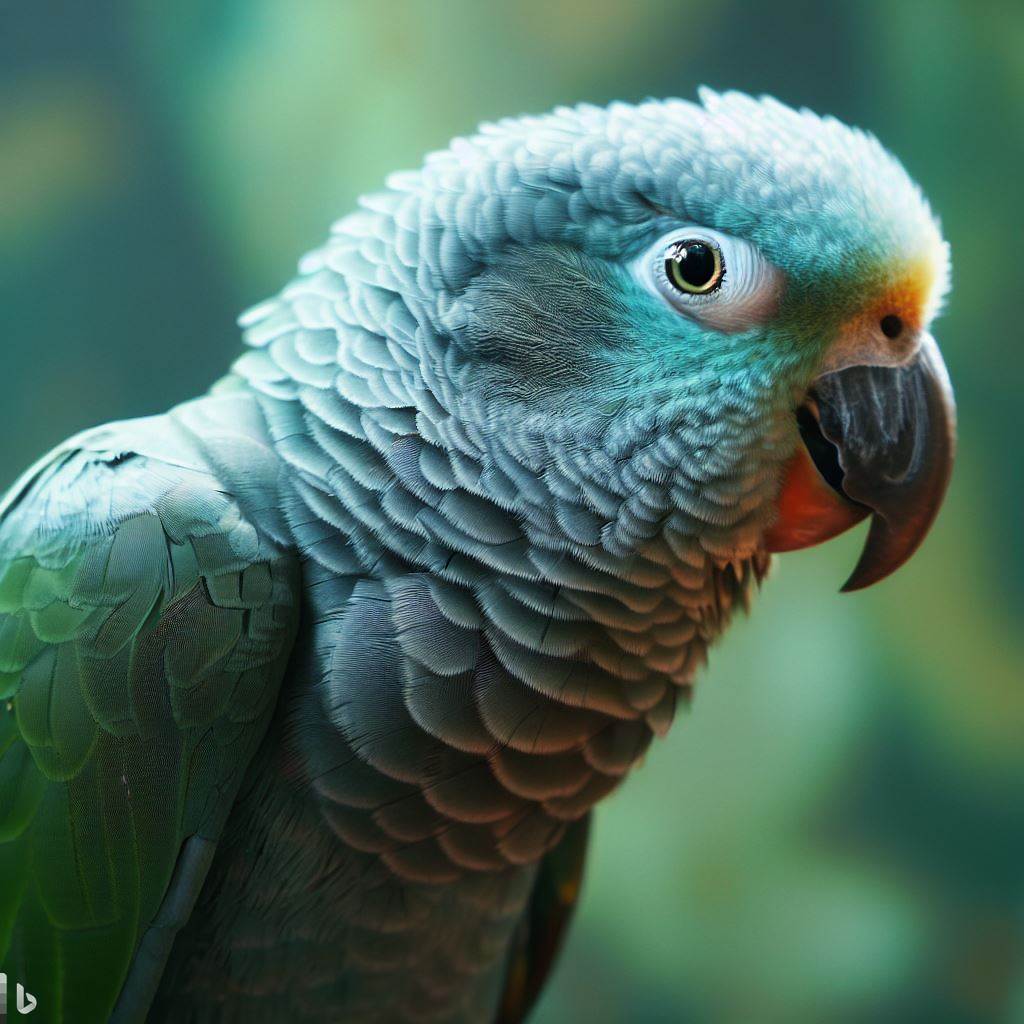A close-up, highly detailed photograph of a tropical parrot dominates the frame, with the bird taking up approximately three-quarters of the image in a clear, profile view. The parrot is set against an out-of-focus, vibrant green and yellow background, adding a lively contrast to the composition. The parrot’s light blue head transitions into darker blue and turquoise hues around its eyes, which feature dark irises rimmed with yellow. 

Above and below the parrot's brown, hooked beak are distinct patches of orange feathers. The partial visibility of the bird’s left wing reveals green feathers, while its trunk feathers gradient from light blue to dark and medium green tones. The detailed textures of the layered feathers are evident, particularly where the bird looks slightly fuzzy atop its head, further emphasizing the intricate beauty of this exotic bird. A barely noticeable watermark appears at the bottom of the image.